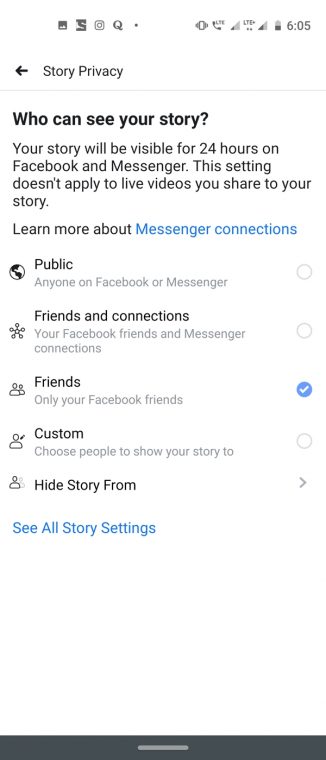The image depicts the "Story Privacy" settings page on Facebook. At the top left corner, there is a Facebook icon indicating the section being viewed. The title "Story Privacy" is prominently displayed at the top, alongside a back button. 

The central text reads: "Who can see your story? Your story will be visible for 24 hours on Facebook and Messenger. This setting doesn't apply to live videos you share to the story." Below this, there is a blue link labeled "Learn more about Messenger Connections," while the rest of the text is in black.

Five selectable privacy options are listed with circular checkboxes: 
1. **Public** - Anyone on Facebook or Messenger.
2. **Friends and Connections** - Your Facebook friends and Messenger connections.
3. **Friends** - Only your Facebook friends. This option is currently selected, indicated by a blue tick mark.
4. **Custom** - Choose specific people to show your story to.
5. **Hide Story From** - Select people to hide your story from.

At the bottom, there is a blue link that reads "See all story settings," attracting attention against the otherwise black text. The page design ensures that the active selection and additional settings are distinctly noticeable, guiding the user through privacy customization for their story.